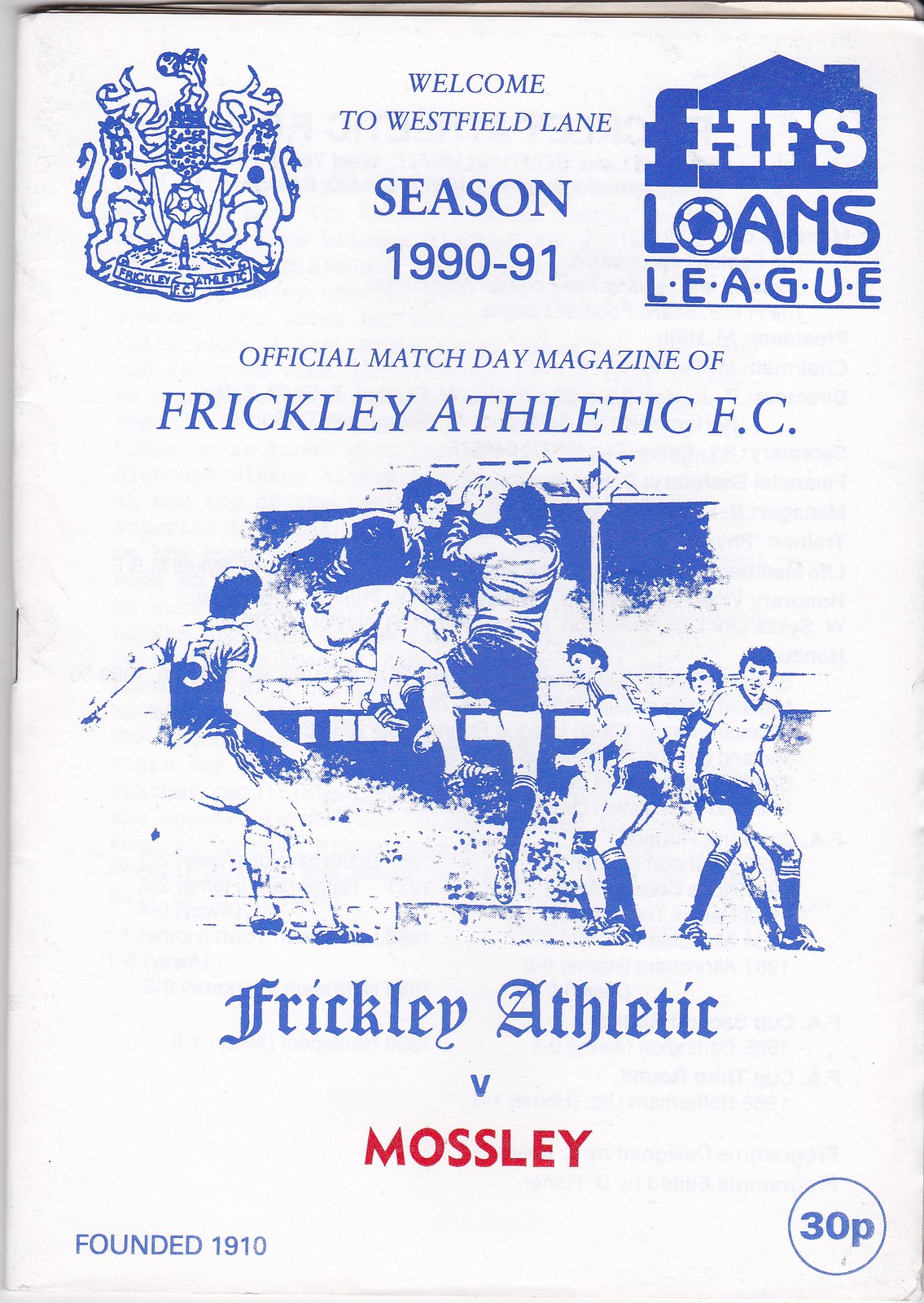The image is the cover of an old magazine, primarily characterized by its white paper and blue ink. At the top, it features the title: "Welcome to Westfield Lane, Season 1990-91 Official Match Day Magazine of Frickley Athletic FC." Prominent logos adorn the top left and top right corners, including a notable coat of arms in the top left. Centrally, there's an image of six people in sports attire, likely engaged in a football (soccer) game, standing or positioned on a field. Below this photograph, text in blue reads "Frickley Athletic vs. Mosley," with "Mosley" highlighted in red. The bottom left corner indicates "Founded 1910," while the bottom right shows "30P" circled in blue. The overall layout positions most of the text at the top and bottom, framing the central image, which may hint at an advertisement for a historical game day or event.